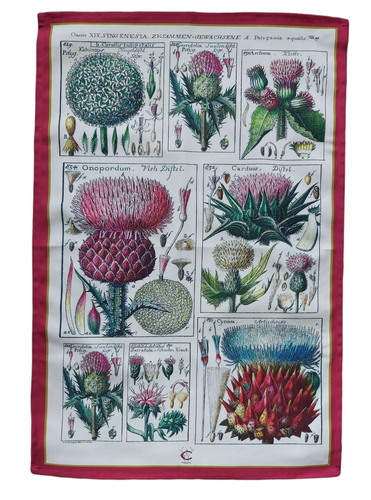This image depicts a vertically rectangular fabric, possibly a scarf or blanket, adorned with a series of botanical illustrations framed by a red border. The fabric showcases nine individual boxes arranged in three rows (three at the top, two in the middle, and three at the bottom) containing detailed, old-school-style drawings of various plants. Central among them is a plant referred to as "stinging meadow," characterized by its thorny stalk, jagged leaves, and a red, frilly top with visible seeds. The top rows feature three distinct plants labeled with Latin words, including a fully green ball-like plant and a red-pink flower with thick leaves. The meticulous depiction extends to showing seeds and intricate details of other plant species, suggesting the diagram's origin from a horticultural or biological reference collection.